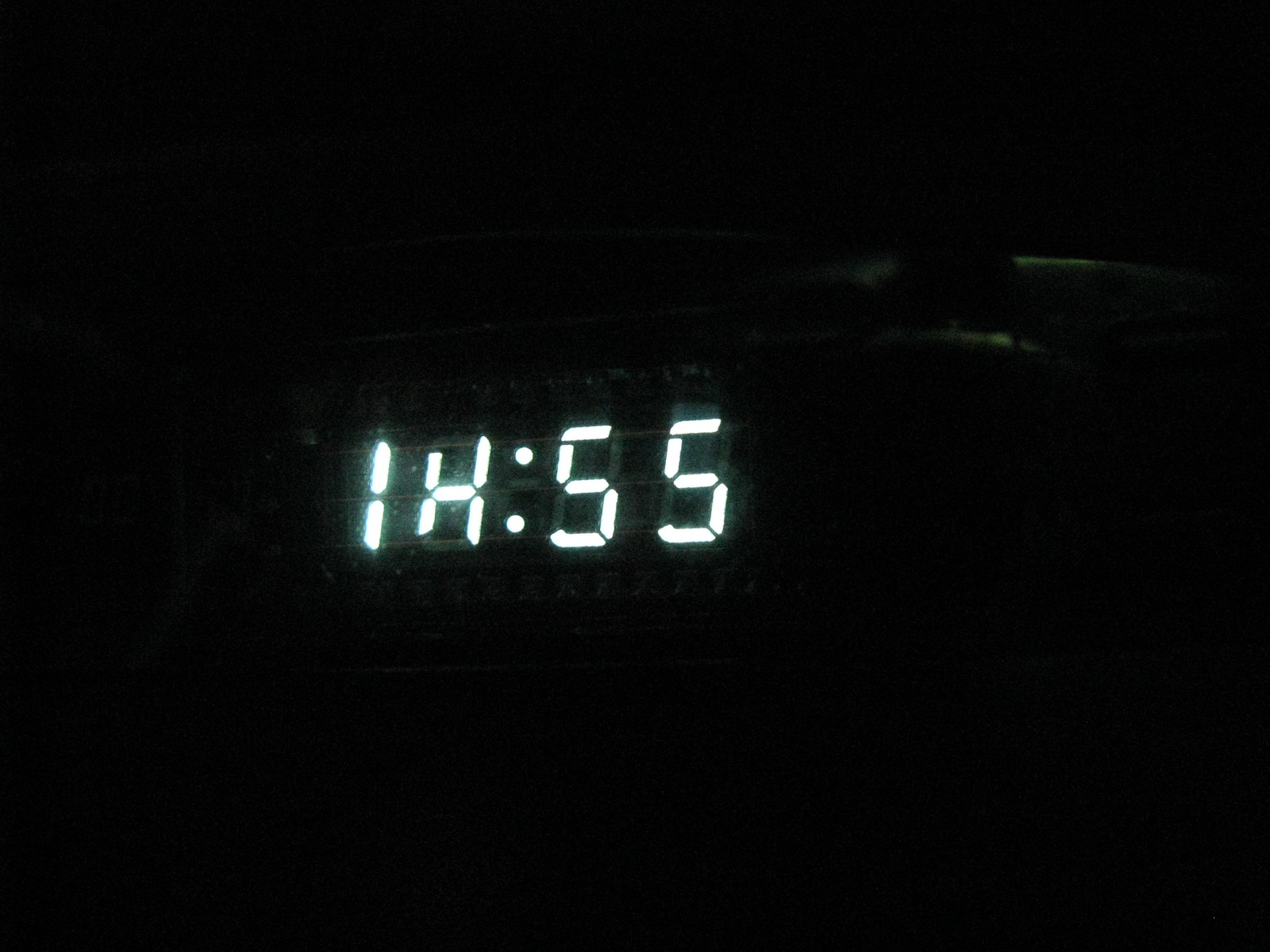This is a photograph of a digital clock or possibly a clock integrated into an appliance, set against a pitch-black background. The display shows the time as 1H:55, where the second digit is irregular and potentially defective, resembling an incomplete or distorted 'H'. The time digits are illuminated in a white color, providing a glowy effect in the darkness. There are some whitish horizontal streaks or reflections in the upper right corner of the image, adding to the nocturnal ambiance. The clock or appliance itself appears to be older, with some debate over whether it is part of a microwave, oven, or standalone device. The partial glimpse of something silver might be a reflective surface on the appliance. The irregular display and surrounding darkness emphasize the clock's damaged state and mysterious setting.